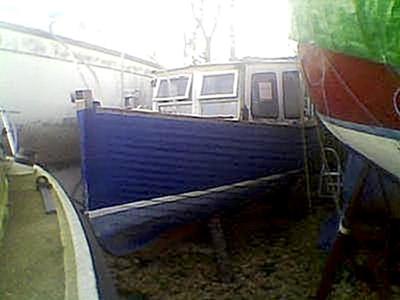The image is a slightly blurry, square photograph taken outside on a bright but cloudy, foggy day. It prominently features several grounded boats resting on stilts. The central boat is mostly blue with a white cabin and cracked-open white-framed windows. To the right, there's a red and white boat partially covered by a green tarp. On the left, a boat with an interior resembling green carpet is visible. The water beneath the boats is murky, littered with brown leaves. In the upper left corner, a stone walkway with a curved edge and a potential bridge can be seen. The background includes some trees and a brightly lit sky, casting a foggy ambiance over the scene. The composition is framed by a few details like open windows and ropes on the boats.